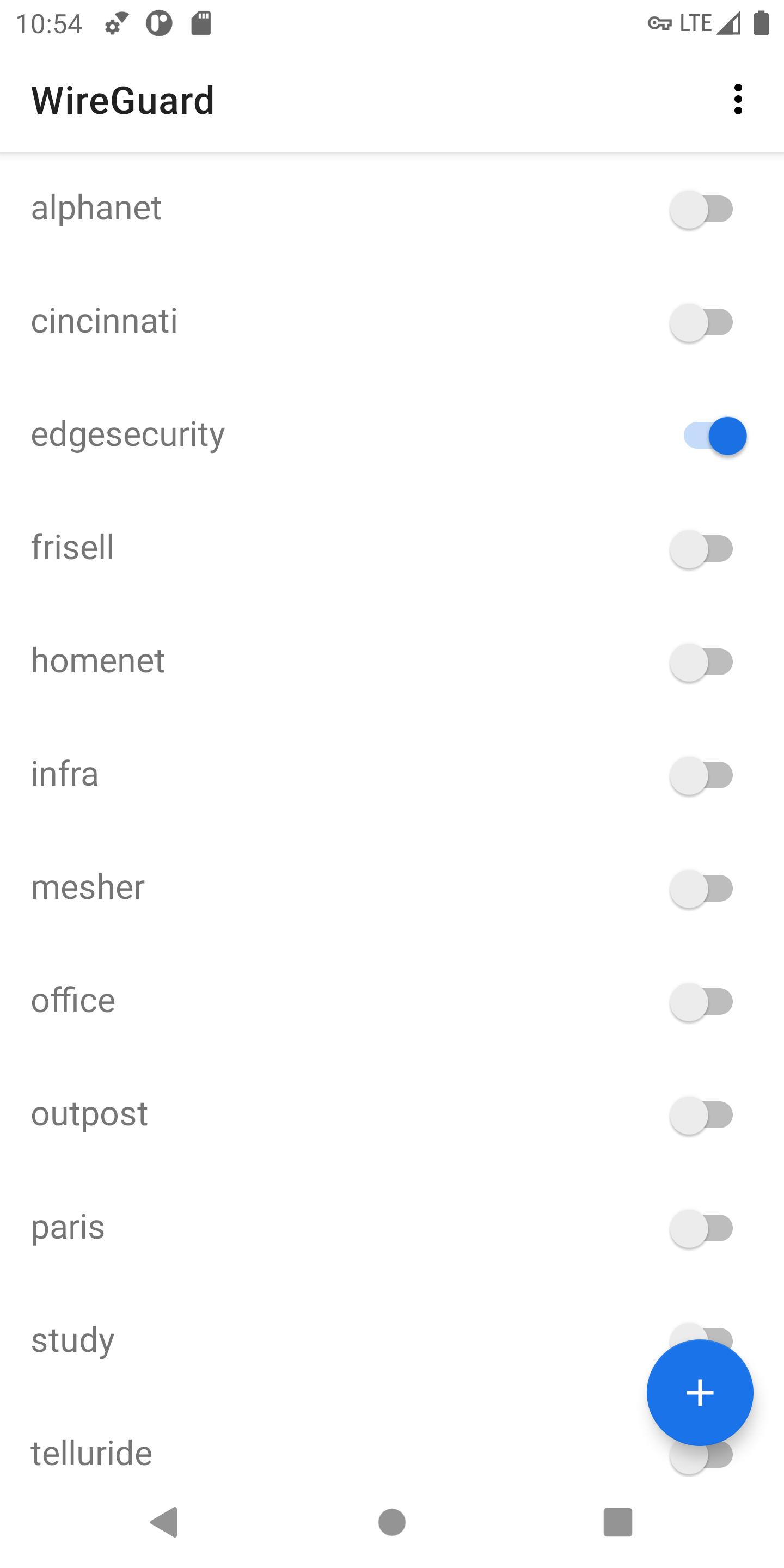This image is a detailed screenshot captured from a phone, displaying a vertical, single-column interface. 

In the upper-left corner, the time "10:54" is visible, while the upper-right corner shows a fully charged battery icon. Directly below, the word "WireGuard" is displayed in bold, accompanied by a three-dot menu icon indicating additional options. An underline separates this header from the remaining content.

The interface then lists twelve rows, each row consisting of a label on the left and a toggle switch on the right. Of the twelve rows, only the third row's toggle switch, labeled "Edge Security," is activated and shown in the "on" position. The names of the rows from top to bottom are as follows: 

1. Alphanet
2. Cincinnati
3. Edge Security (toggled on) 
4. Frizzell
5. HomeNet
6. Infra
7. Mesher
8. Office
9. Outpost
10. Paris
11. Study
12. Telluride

At the bottom of the screen, there are three dark gray navigation icons: a back arrow, a circle, and a square. Additionally, located to the upper right of the gray square is a blue circle with a white plus sign, indicating an option to add more applications.

The image effectively highlights that only the "Edge Security" application has been activated under the "WireGuard" list, with all other applications remaining off.